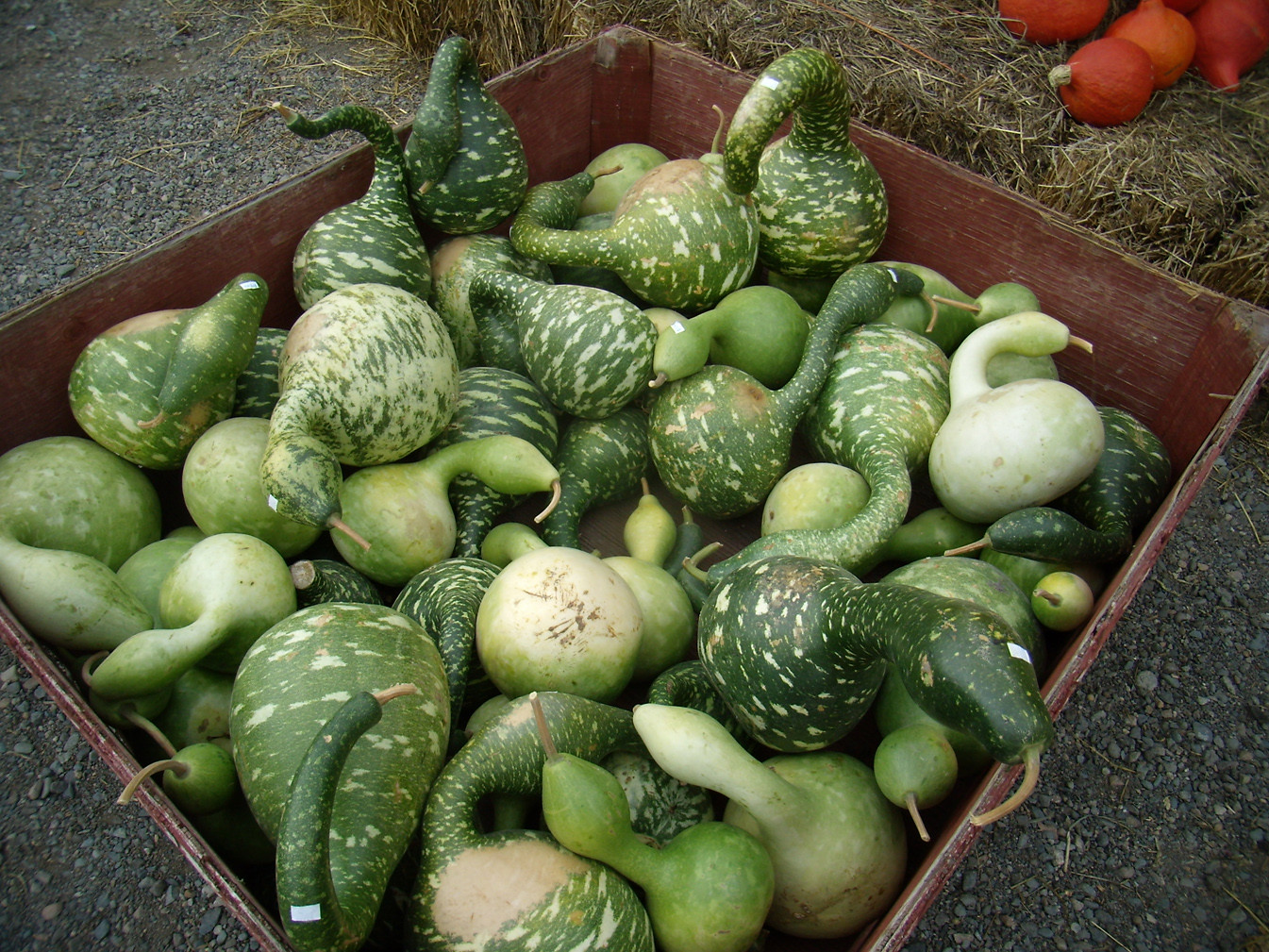This is a zoomed-in image of a reddish-brown wooden crate containing an assortment of squash and other vegetables. The vegetables inside the crate display a variety of shapes and colors: some are light green with a brown stem, some are dark green with white stripes, others are predominantly white with green stripes, and a few appear bruised with brown patches. The squash are irregularly shaped, with many having long, curved necks resembling swans. The crate is situated on a gravel and dirt surface. In the upper right corner of the image, partially obscured, are hay bales and deep orange pumpkins, suggesting a farm setting.